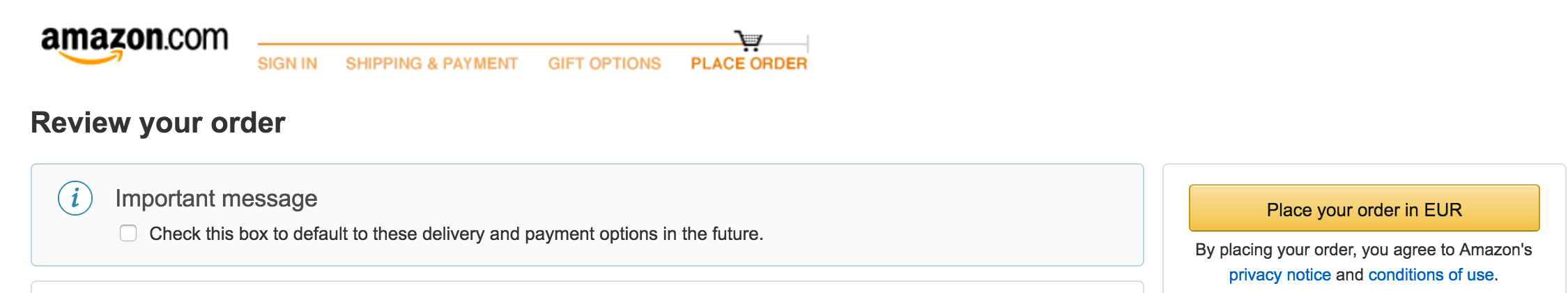The image depicts a webpage from Amazon.com showcasing a typical checkout screen. At the top, it clearly states "Amazon.com" next to the familiar curved arrow logo. Below this, the user is prompted to "Sign in," followed by sections for "Shipping and Payment," "Gift Options," and "Place Order," all highlighted in Amazon's characteristic orange color.

The central section of the page displays "Review your order" with an "Important Message" enclosed in a gray box, advising users to check a box to set these delivery and payment options as defaults for future purchases. To the right, it includes an option to pay in EUR (Euros), and a reminder that by placing the order, the user agrees to Amazon's Privacy Notice and Conditions of Use. These latter terms are clickable links presented in blue text.

A prominent gold bar labeled "Place your order" is positioned as the cell to finalize the purchase. The overall text varies slightly in font, creating a somewhat disjointed appearance. The bottom part of the image is cut off, indicating there are additional elements not visible in the screenshot.

This image encapsulates a typical step in the Amazon online shopping process, providing a detailed look at the final steps before order placement.